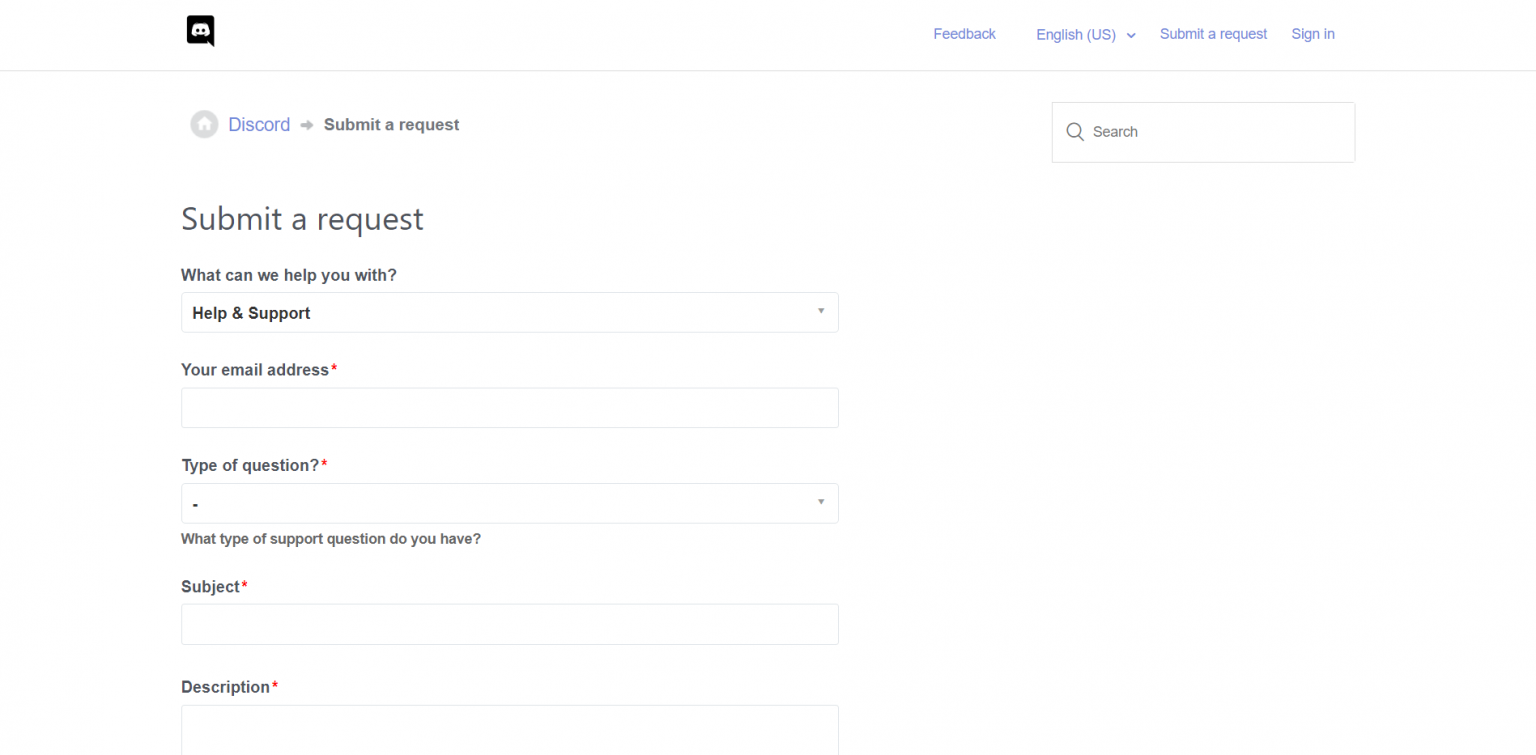This image displays the Discord "Submit a Request" webpage in detail. In the upper left corner, the recognizable Discord logo is prominently featured. Directly below it is a home icon, followed by a link labeled "Submit a Request" with a right-pointing arrow, indicating the current active page.

The webpage itself features a clean, white background with light black text. The header of the page reads "Submit a Request," accompanied by a prompt asking, "What can we help you with?" Below this, there is a dropdown menu currently set to "Help & Support."

Further down the form, the mandatory field labeled "Your email address" is marked with a red asterisk. Following this is another required field, "Type of question," also accompanied by a red asterisk, featuring a dropdown menu for selection.

Underneath, the section asks, "What type of support question do you have?" which is followed by another mandatory field labeled "Subject." Below the subject field, there's a larger text area for elaboration, labeled "Description," also marked with a red asterisk.

In the upper right corner of the page, there is a search box for navigating the site. Just above this, there are additional links for feedback, a language selection dropdown menu currently set to "English, U.S.," and options to either submit the request or sign in.

This comprehensive layout ensures users can easily navigate and provide the necessary details for their support requests on the Discord platform.